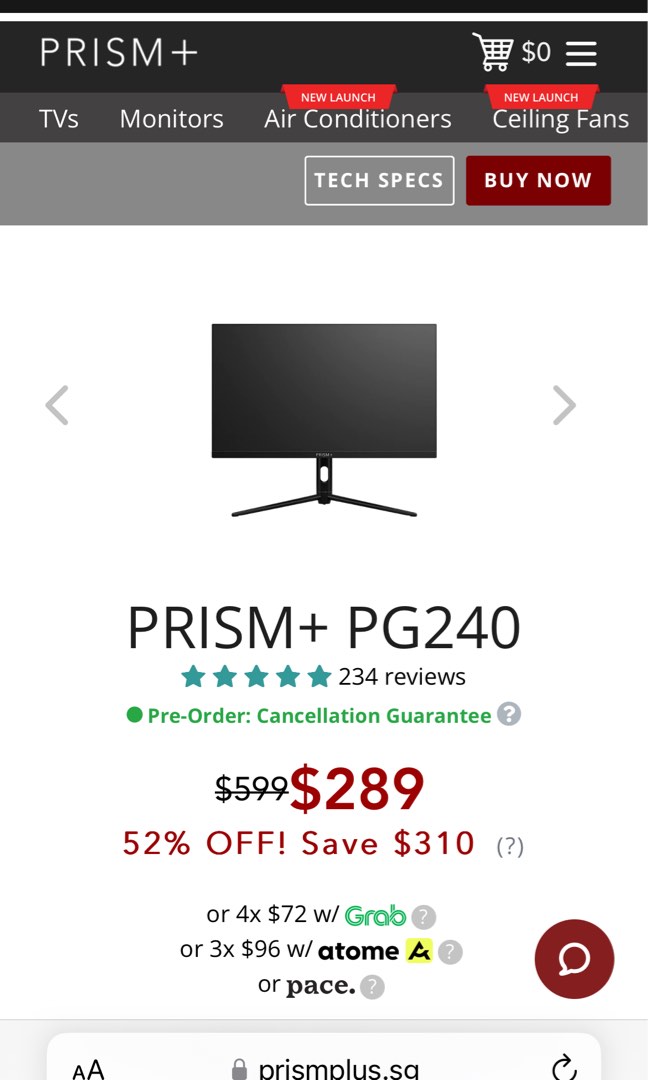The image depicts a smartphone screen showcasing an e-commerce app with a TV listed for sale. The top section of the screen features the brand name "Prism Plus," a shopping cart icon indicating a zero-dollar balance, and a tab menu against a black background. Directly below this is a navigation bar with four categories: "TVs," "Monitors," "Air Conditioners," and "Ceiling Fans." A "New Launch" label with a bright red background is placed above the latter two categories.

Further down, the section displays a flat-screen TV named "Prism Plus PG240" positioned on a stand with navigational arrows on either side of the TV image to browse through additional photos. Accompanying the TV image are product details: out of 234 reviews, the rating stars are shown in blue. The phrase "Pre-order cancellation guaranteed" appears in green text. The previous price of $599 has been slashed to $289, reflecting a 52% discount and saving of $310, highlighted in red text.

Additional purchase options are presented below the price, alongside a dark red circle housing a chat icon on the right-hand side. The bottom of the screen shows the website URL, "prismplus.sg," flanked by a refresh icon on the right and dual "Aa" icons on the left. The background of the screen is predominantly white, providing a clean contrast for the detailed information displayed.